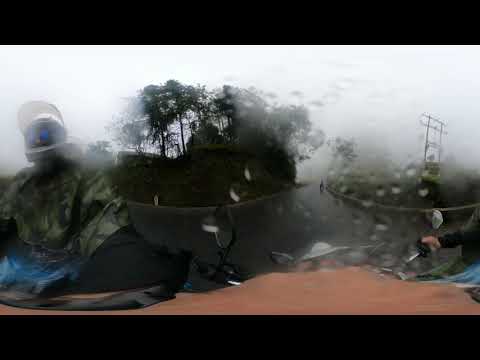The image captures a rainy, misty day outdoors, seemingly taken from a GoPro. The lens is speckled with water droplets, contributing to the overall blurriness. In the center of the frame, distant trees reach into the gray, foggy sky, adding depth to the scene. On the right side, an electric pole and a small yellow sign can be discerned. A figure stands on the left, facing the camera, clad in a camo poncho and a white motocross helmet with a clear visor. This person is wearing sunglasses and is near what appears to be a wet, slick road. The foreground hints at a biking adventure, as we see handlebars and another individual's hand, outfitted in a long-sleeved black top, gripping them. The disorienting nature of the image and the cloudy, rainy weather envelops the entire scene, making it difficult to capture finer details.